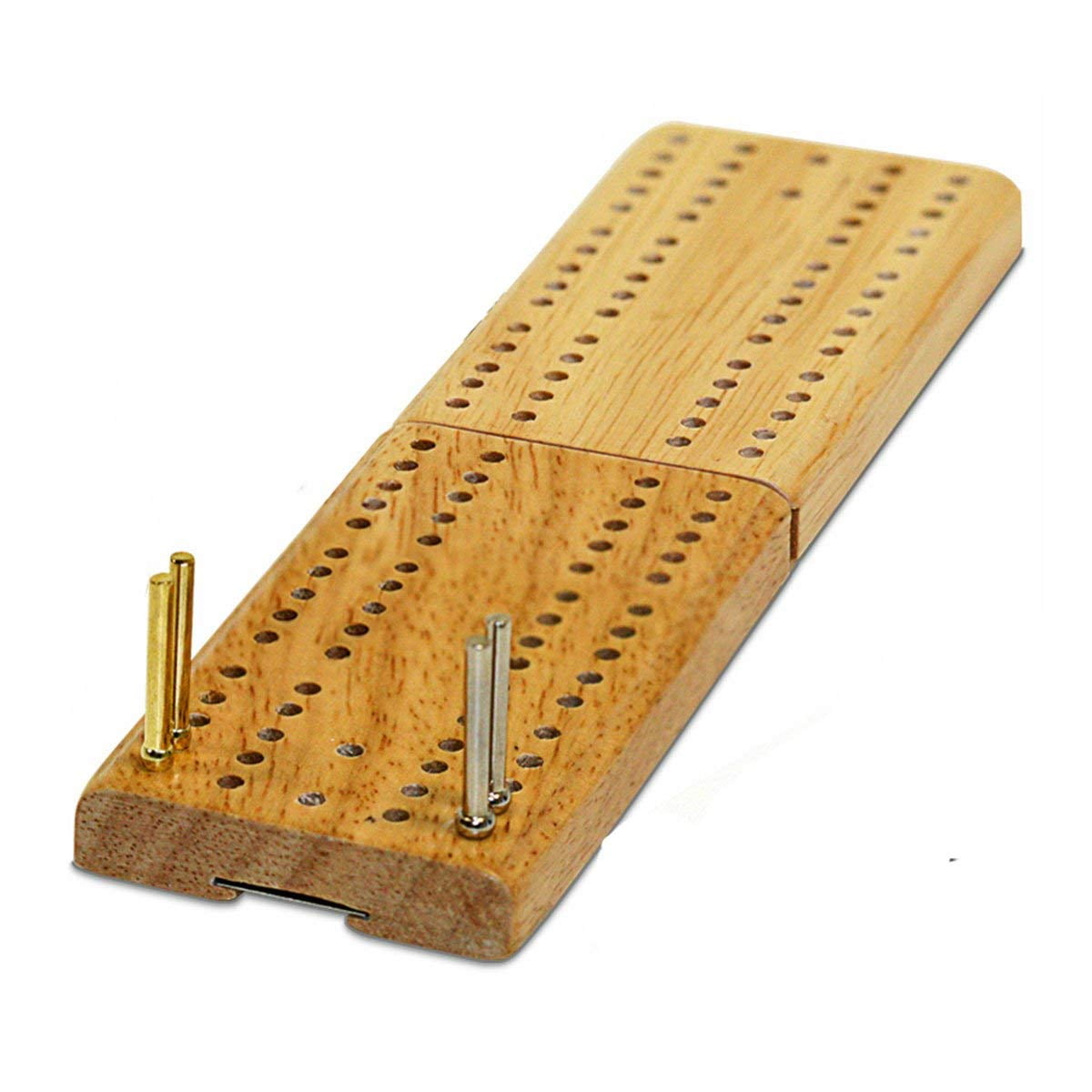The image depicts a cribbage board positioned against a white background, viewed from an angled perspective that stretches from the bottom left to the top right. The board consists of two wooden sections; the lower, darker section pointing to the left, and the higher, lighter-toned section pointing to the right. Both sections share a medium wood tone, likely resembling honey oak. Notably, the lower board features four vertical pegs: two gold on the left and two silver on the right. Additionally, an open area beneath the bottom center of the darker section reveals a small card nestled within it. The cribbage board's holes are drilled in four parallel lines, emphasizing the board's structured design.